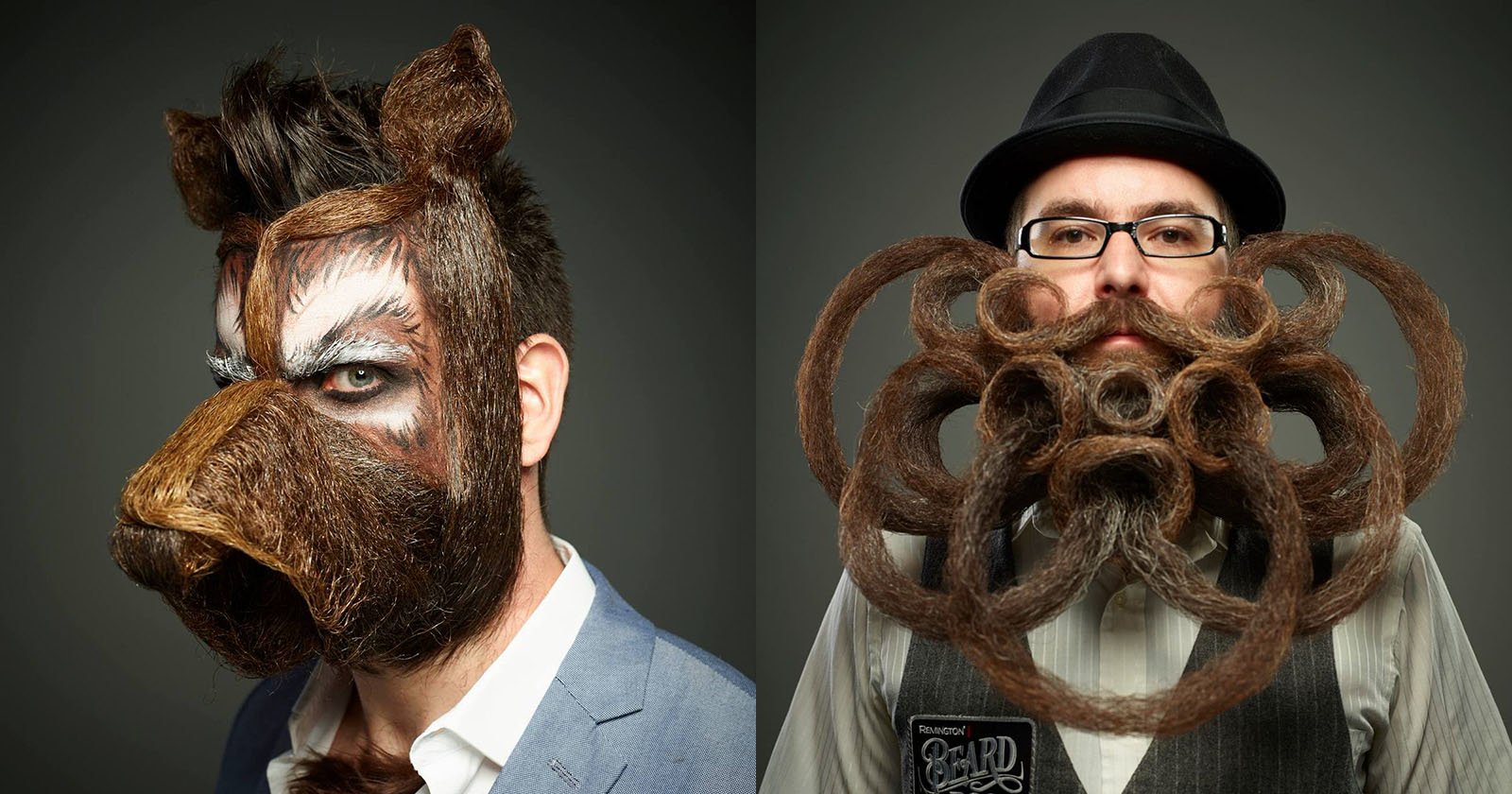This surreal, full-color composite photograph, set against a plain gray background, showcases two ingeniously altered portraits of Caucasian men, both indoors. On the left, a man in a blue suit and white shirt features a bizarre, photoshopped transformation where his face resembles a brown-furred dog, complete with a muzzle-like extension across his nose and cheeks, fur covering his ears and neck, and blue eye makeup accentuating the surreal appearance. To the right is another man wearing a black pork pie hat, dark blue glasses, a gray vest with the text "Farmington Beard" on it, and a white striped shirt. His facial hair is extraordinarily styled, consisting of multiple handlebar mustache strands radiating outward and looping around his face from his cheekbones down to his mid-chest, forming intricate concentric circles. This dual-image composition marvelously combines photographic realism with fantastical, meticulously detailed alterations, creating an extraordinarily bizarre and thought-provoking piece.